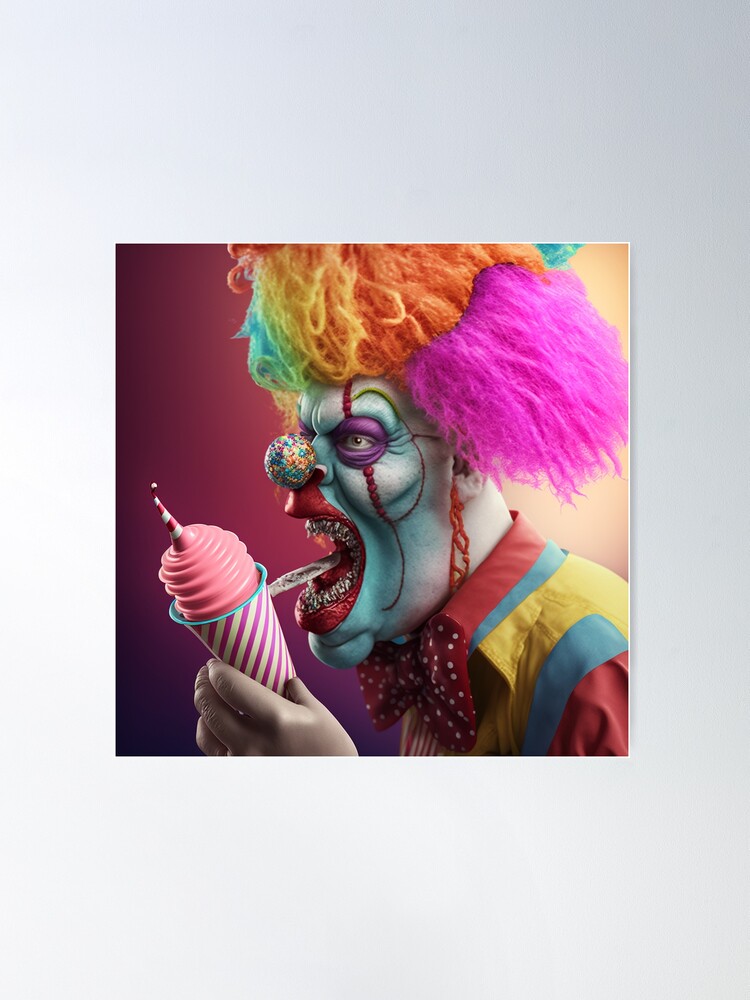This detailed digital image showcases a terrifying clown adorned in an array of bright, vivid colors. The clown faces the left side of the image, with piercing, metallic silver teeth visible through its open mouth. Its hair, resembling cotton candy, bursts with shades of pink, yellow, orange, and green; the green, yellow, and orange strands stand straight up, while the pink strands hang down, adding to its wild appearance. The clown's skin is an unsettling green, and its nose is a sequined, multicolored sphere. Eye makeup, outlined in purple, is accentuated by red jewel lines extending down from the centers of its eyes and further adorned with red chain-like details descending from its ears.

The background radiates in red and yellow, complementing the clown's colorful attire. It sports a flamboyant shirt with a vividly detailed collar transitioning from red to green and yellow, with hints of blue fabric above the red sleeves. The clown’s attire is completed with a red and white polka-dotted bow tie, adding to the chaotic color scheme.

In its left hand, the clown holds a purple and white striped cup containing pink ice cream, whimsically topped with a mini clown hat that ends in a bell. There appears to be a confusing gray and white element resembling either a spoon handle or the clown's tongue extending from the cup to its mouth. The clown's hand is unnaturally gray, likely a stylistic choice emphasizing its eeriness. The overall composition, marked by vibrant hues and unsettling features, creates a disturbing yet compelling visual narrative.